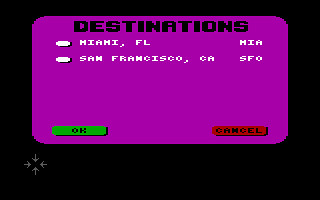The image showcases a small screenshot of an application screen with a predominantly black background. Centered on the screen is a purple rectangle with curved edges, adding a smooth and modern touch to the interface. At the top of this rectangle, the word "Destinations" is prominently displayed in black text. Below this heading, white lettering lists actual destinations.

To the far right of the text listing Miami, Florida, there is a white oval containing "MIA," serving as the airport code for Miami. Similarly, next to the text listing San Francisco, California, is another white oval with "SFO," its airport code. The rectangle further features two distinct buttons at its bottom corners: a green rectangular "OK" button on the bottom left and a red rectangular "Cancel" button on the bottom right, providing clear options for user interaction.

Additionally, on the bottom left corner of the overall black background, there is a centered arrow design pointing up, down, left, and right, forming a crosshair-like pattern, likely intended for navigation or adjustment purposes. The combination of these elements suggests a carefully designed user interface for choosing travel destinations.